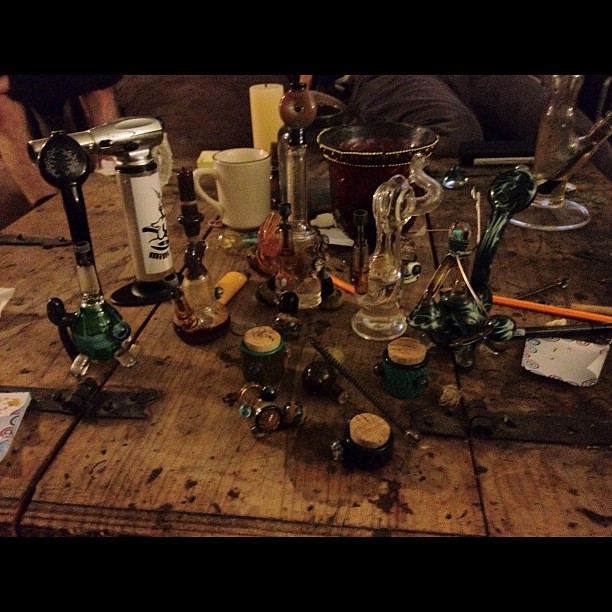This photograph captures a cluttered, low, old-looking wooden table, possibly a repurposed door, covered with a variety of smoking paraphernalia. Various devices, including pipes and bongs of different shapes, sizes, and colors, are spread across the surface. Several tall candles and a light beige coffee cup are also present on the table, which shows significant signs of wear, including burn marks. Among the collection are small jars with cork tops, a business card, a blowtorch, a brass or bronze bucket, and a hurricane lamp in the background. Additionally, a dark reddish-colored glass with a beaded rim stands out at the center of the table, surrounded by green and clear twisted glass items. Scattered pencils complete the scene, while the legs of people seated on a sofa can be seen behind the table. The overall impression is of a dimly lit setting with an assortment of drug paraphernalia and related items.